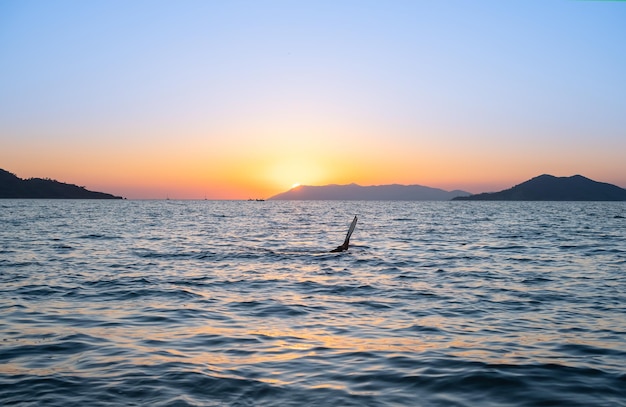In the foreground of this captivating image lies a vast, tranquil ocean under an evening sky. The water, gently rippling with modest waves, hosts a mysterious protrusion at its center, potentially a blackbird’s wing as it dives in search of prey. In the background, a dramatic sunset paints the horizon with a gradient of colors, transitioning from deep blue at the top, through vibrant oranges and yellows near the barely visible sun, to soft pink hues reflecting on the water's surface. Framing this serene scene are low-lying hills and small mountains on either side, with an imposing, shadowy mountainous landform in the distance, accentuating the natural beauty of the setting sun. The sky above is clear, giving way to this split canvas of day blending into night.